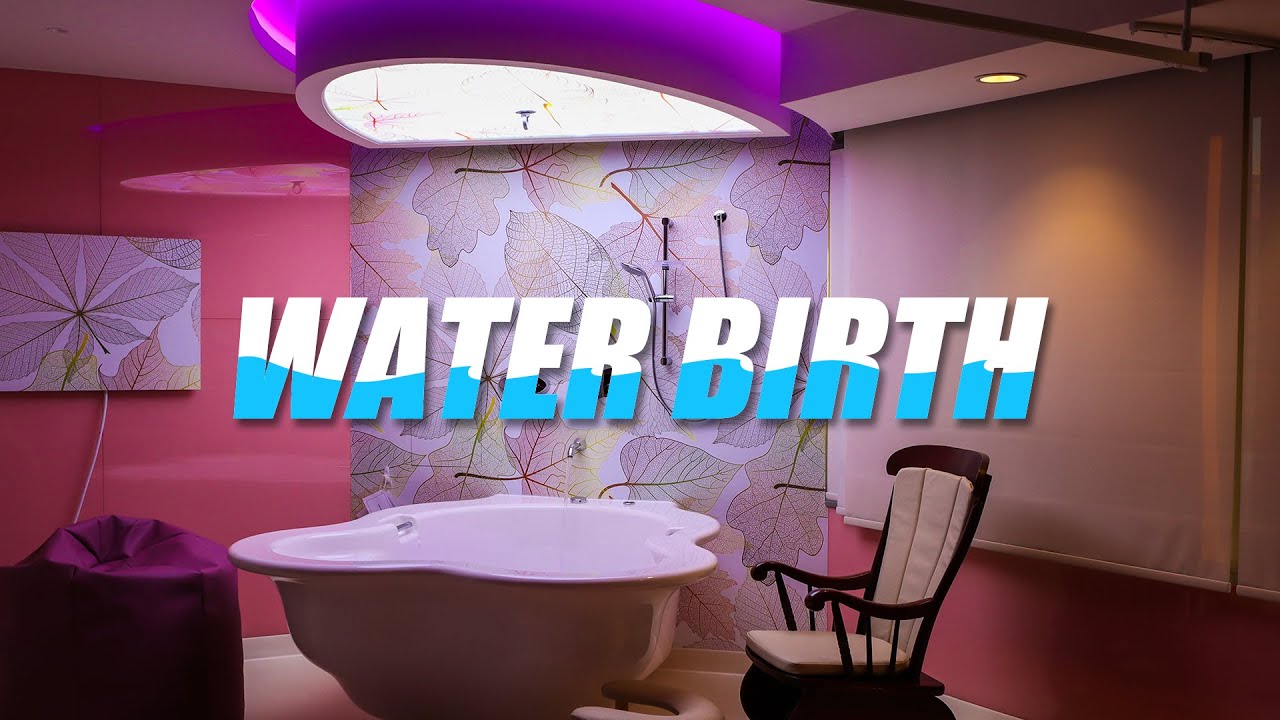The landscape-oriented image features white and blue italicized text in the center that reads "WATER BIRTH." The top half of the text is white, while the bottom half is blue with a wave-like design. The scene depicts a brightly colored room that appears to be part of a promotional material focusing on water births. The room has various shades of pink walls and ceiling, with one wall beautifully painted with leaves in green, yellow, and pink hues. On the left wall, there is an art piece featuring a white background with leaf designs. 

Dominating the center of the room, directly below the text, is a large white, freestanding tub designed to accommodate water births. To the right of the tub is an antique-style wooden rocking chair with white cushions. On the left side, there's a maroon-colored bean bag. The ceiling features specialized lighting that includes neon and possibly purple hues, providing a unique ambiance. A closer inspection reveals a faucet with water flowing into the tub, emphasizing the water birth theme. Overall, the room combines elements of comfort and utility with an eclectic design that includes wooden furniture and modern lighting, aiming to create a nurturing environment for the birthing process.